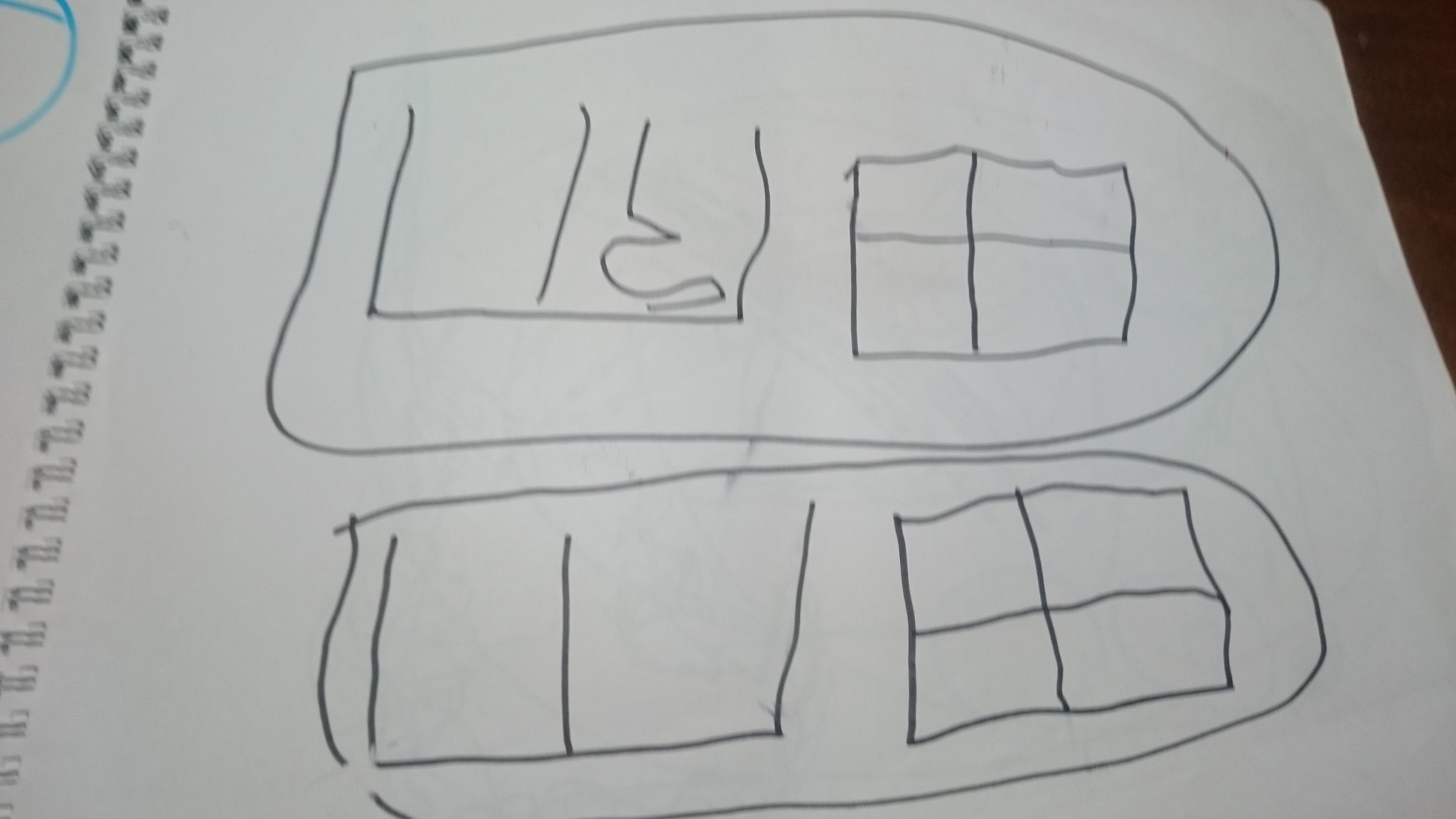This sketchbook page appears to be from a child's collection, featuring two distinct drawings, each contained within an oval frame with a slightly flattened left side. 

In the bottom oval, there is a large, upside-down letter "E." Notably, the middle stroke of the "E" is as long as the top and bottom ones, resulting in a shape that resembles side-by-side open containers, or an "E" lying on its back. Adjacent to this is a simpler, yet imperfect, rendition of a classic four-pane window, akin to a window intersected by a big plus sign.

The top oval mirrors the bottom one with some slight variations. Here, the upside-down "E" is slightly larger, and within the lower part of the rightward box-like section of the "E," there is an additional scribbled shape resembling an "S" with a division sign above it. The enclosing oval for this drawing is also larger than the one below.

These whimsical and imaginative sketches capture the innocent and exploratory nature of childhood art.